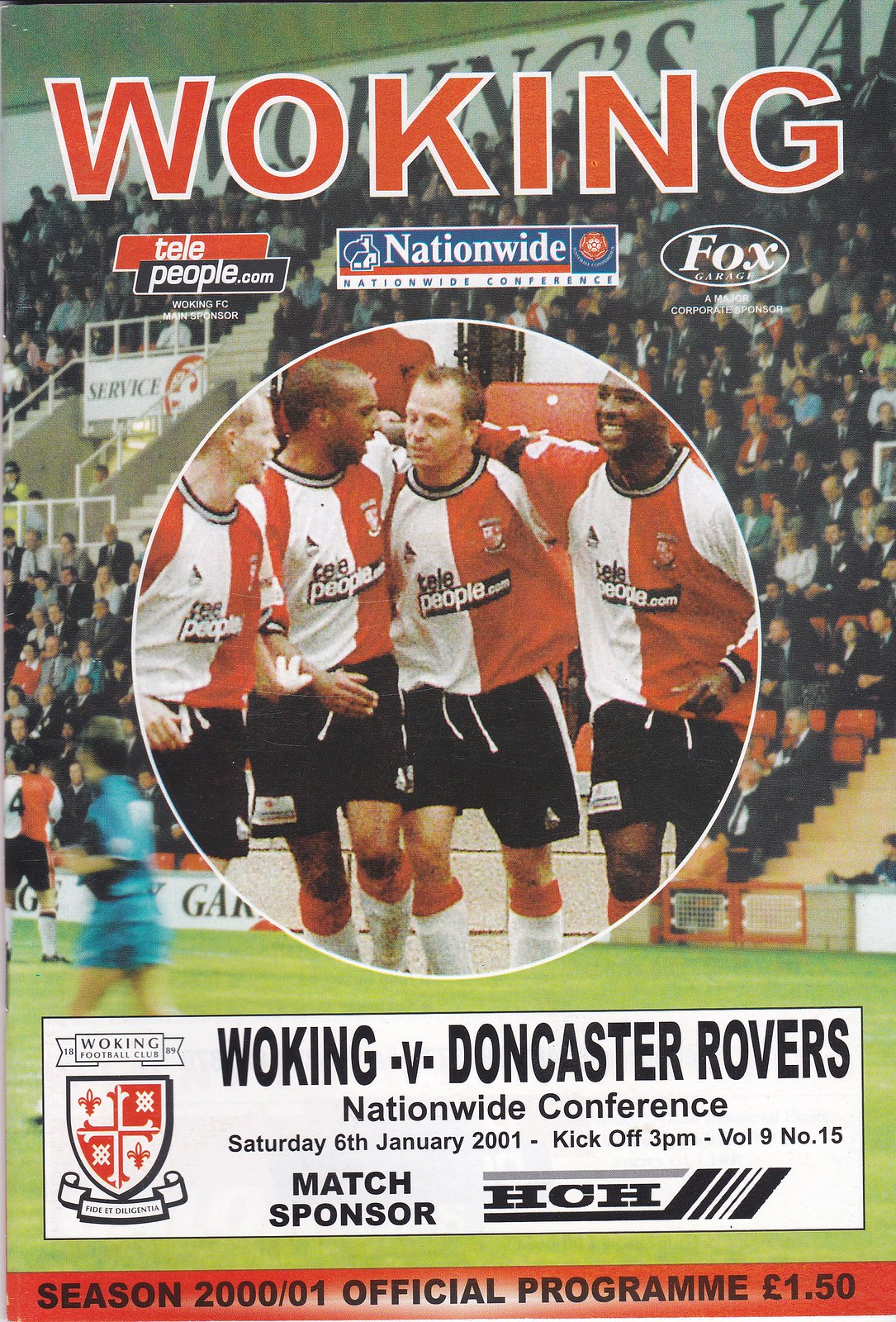This detailed and colorful cover of a soccer program for Woking Football Club features the bold title "WORKING" in orange letters with a white outline prominently placed at the top. The background showcases a packed stadium teeming with fans, creating an energetic atmosphere. Just beneath the main title, three sponsor logos for Telepeople, Nationwide Conference, and FOX are aligned. Dominating the center of the cover is a large circular photograph of four soccer players—two black men and two white men—each wearing a uniform with an orange section on the right and a white section on the left, paired with black shorts. These players are standing with their arms around each other, focusing inward.

Encircling the central image, key details include the website "TITLE OF PEOPLE DOT COM." Below the circle, a white rectangular box provides crucial match information: 
"WORKING V. DONCASTER ROVERS 
NATIONWIDE CONFERENCE 
SATURDAY 6 JANUARY 2001 
KICKOFF 3 PM 
VOLUME 9 NUMBER 15 
MATCH SPONSOR HCH."

On the left side of this box, a ribbon inscribed with "WORKING FOOTBALL CLUB" tops a badge-shaped decal containing red characters. Across the bottom of the cover, a red strip features black text announcing, "SEASON 2000-01 OFFICIAL PROGRAM £1.50." The entire design, printed in vibrant color, embodies the excitement and professionalism of the Woking Football Club's official publication.